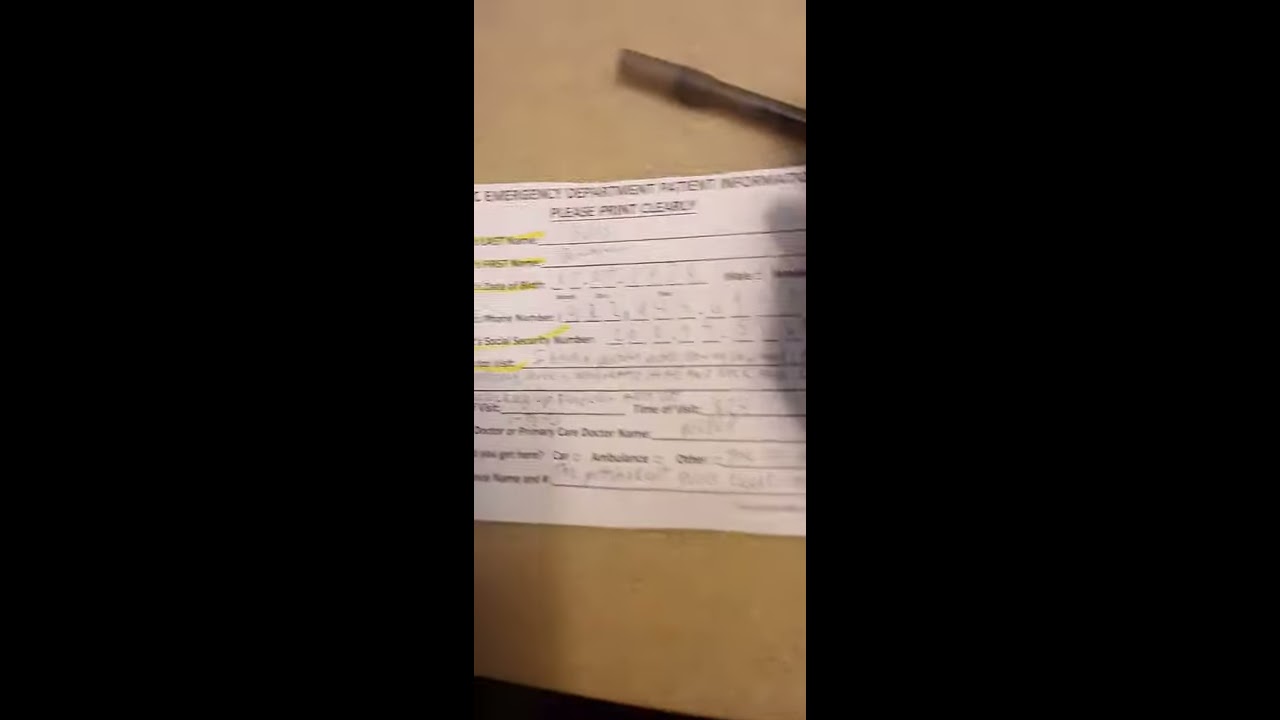The image depicts a slightly blurry scene set on a tan, possibly wooden, rectangular table. At the center of the image lies a white sheet of paper, identified as an emergency department patient information form. Despite the blurry nature of the image, the prominent headings on the form, such as "emergency department patient information" and "please print clearly," can be discerned. The form includes sections for last name, first name, social security number, and phone number, with blank spaces provided for these details, though the actual handwritten information is too faint to read. Positioned in the upper right-hand corner of the scene, there is a black ink pen. The overall setting appears to be indoors, likely within a medical facility such as a hospital. The background colors in the image include shades of brown, gray, black, and white, contributing to the overall neutral tone of the setting.